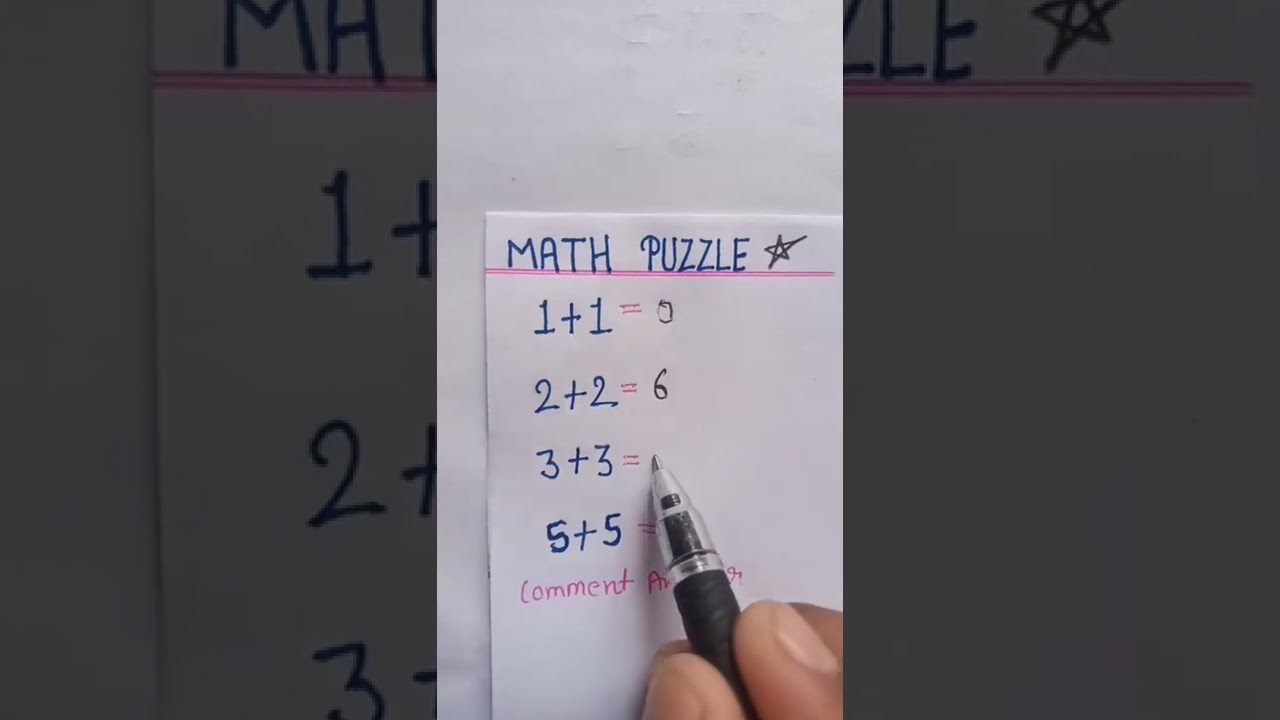In the image, there are multiple pages with the main focus being on a math assignment with the title "Math Puzzle." The title is written in bold blue capital letters with a black star next to it. Below the title, several math equations are listed in blue: "1 + 1" with the answer "0" in black, "2 + 2" with the answer "6," "3 + 3," and "5 + 5". Following these equations, there is a prompt in pink letters that says "comment." The paper with these equations is layered on top of another sheet that partially covers a background where a large blue "MAZZLE" and a red line can be seen. The scene includes a person's hand holding a black pen at the bottom right of the image. The overall color scheme of the image includes white, blue, pink, black, and tan, suggesting it might be a scanned or photographed document viewed on a mobile device.